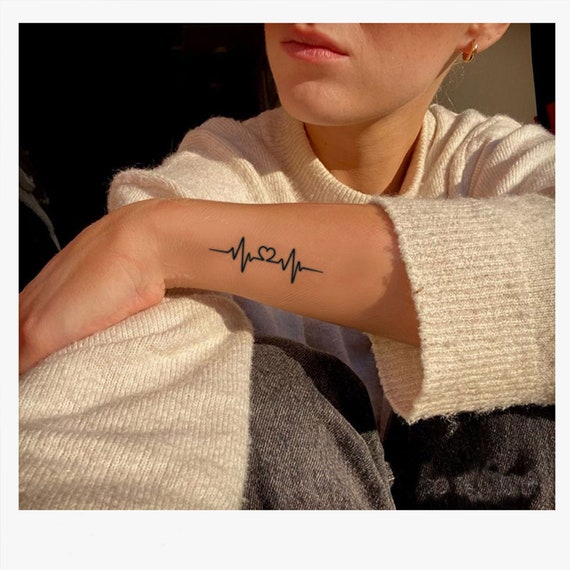This photograph features a close-up of a person in a sitting position, likely a Caucasian female in her late 20s. The image is cut off just below the nose and above the ear, providing a partial view of her face and some of her upper body, along with a bit of her knee. She is dressed in a cream-colored sweater and dark-colored pants, which might be black or dark grey-blue. Her knees are pulled up to her chest, and her arms are crossed, with her left arm draped over her right. 

On the left wrist, there is a black tattoo depicting an electrocardiogram (EKG) line with a heart in the middle. She is wearing a gold earring in her left ear. The background is predominantly black, though there's a cream-colored area on the right side. Sunlight is filtering in, highlighting parts of her body and clothes, adding dimension to the image.